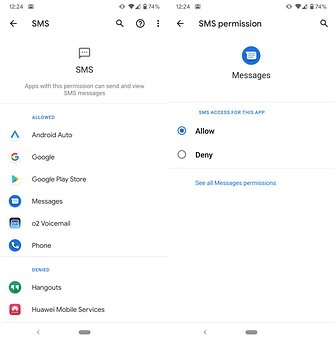The image features two screenshots from smartphones presented side-by-side against a plain white background. The image itself is slightly taller than it is wide, with roughly a 10% difference in height to width ratio.

At the top of each screenshot, the time displayed is 12:24. An unfamiliar icon is present on the upper left, while familiar icons for battery life, signal strength (both cellular and Wi-Fi), are located on the upper right.

Both screenshots display a left arrow in black, the text "SMS," and a magnifying glass icon on the right-hand side. However, the left screenshot includes additional elements: a question mark icon and three vertical dots (indicative of a menu). Below these elements, the left screenshot features a black chat bubble with the text "SMS" centered beneath it. In contrast, the right screenshot displays a blue chat bubble labeled "Messages."

Further down in the screenshots, a series of app icons are visible. The left screenshot contains approximately eight app icons. Meanwhile, the right screenshot prominently features "Allow" and "Deny" options, indicating a permissions prompt.

The differences between the two images highlight varied interfaces and functionalities related to messaging apps and permission requests.